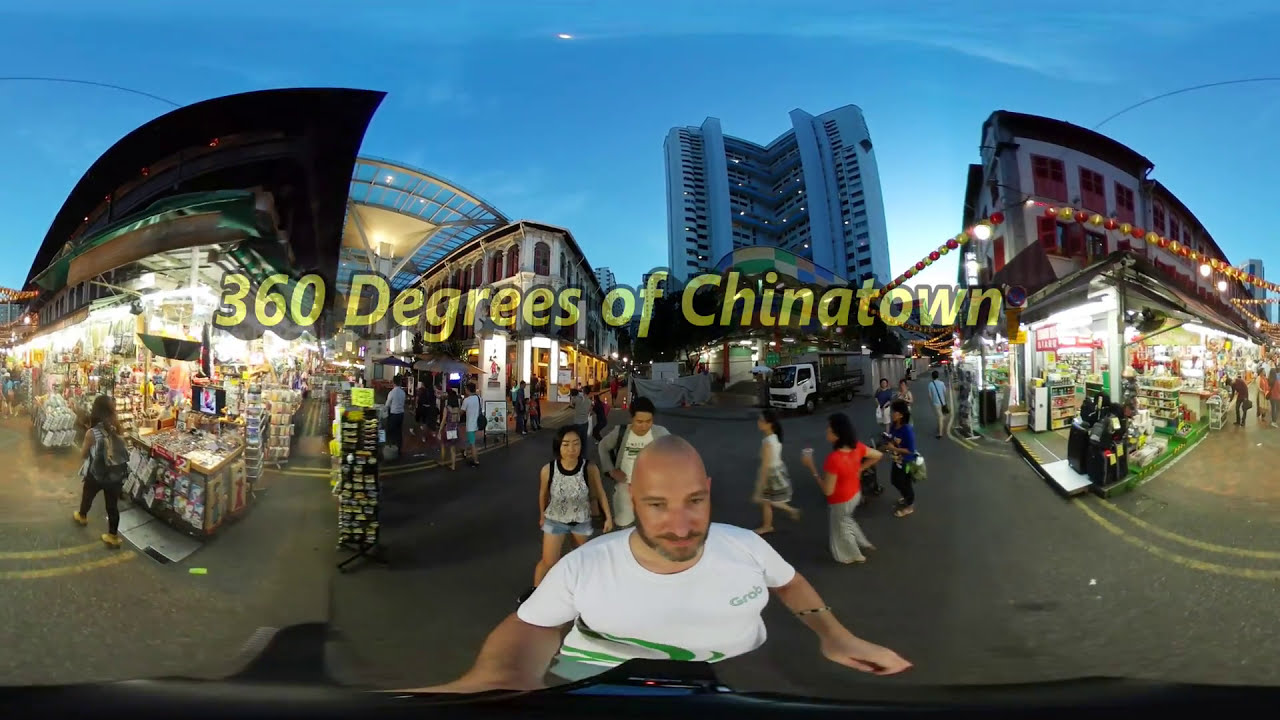This image captures a panoramic view of Chinatown, seamlessly, or perhaps imperfectly, merging three photographs, evidenced by slight curvatures and mismatches in the blue sky overhead. The photo features a bustling evening scene, illuminated by various lights against the darkening sky. The focal point is a bald man of Caucasian descent, prominently positioned in the foreground, wearing a white short-sleeved t-shirt with green print that seems to read either "grab" or "grob." He sports a graying mustache and beard. 

To the left, there's an open-air market, characterized by a completely open storefront without doors, allowing direct access to the products on display. Above the shopfront, a large black sign casts a shadow. A person is seen walking away, intently looking at the storefront items.

The center of the image showcases a mix of architectural heights, including a tall building and lower structures. A truck is parked on the road, where people, likely tourists, walk along black pavement marked with yellow lines, exploring booths that line the streets.

On the right side, an additional open-style shop is noticeable at a corner, adorned with a row of yellow and red bulb lights above it. Behind this shop, there is a two or three-story apartment building. Scattered around are various individuals of Asian descent, contributing to the vibrant street scene.

Spanning the midline of the photo in slightly transparent yellow print with black shadowing, the text "360 degrees of Chinatown" declares the encompassing nature of this panoramic snapshot.